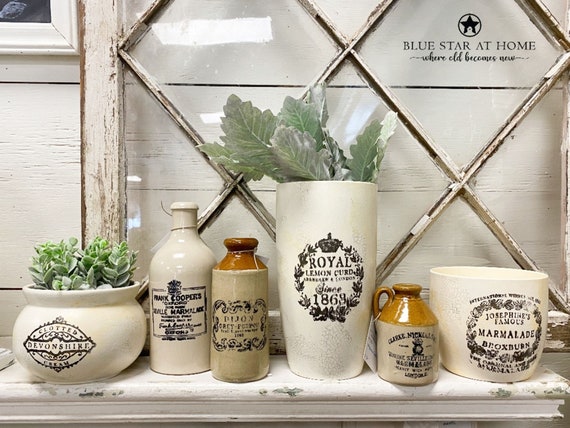This indoor scene appears to be set in a weathered, white wooden room with a vintage aesthetic. Against the backdrop of a glass window featuring diamond wood frames, a white shelf holds an assortment of items, including various bottles and jars. Notably, these containers include a jar of "Royal Lemon Curd" from 1868, "Josephine's Famous Marmalade," and others bearing a "Blue Star at Home" insignia. The collection also includes a series of white and brown bottles as well as larger white vases, some adorned with a black logo, filled with green plants and succulents. The color palette predominantly features muted tones such as beige, light brown, pale green, and peeling white and black, contributing to the aged, rustic charm of the room. The positioning of objects, with bottles and vases on the shelf and plants sprouting from various pots, adds to the overall homely yet nostalgic atmosphere of the space.